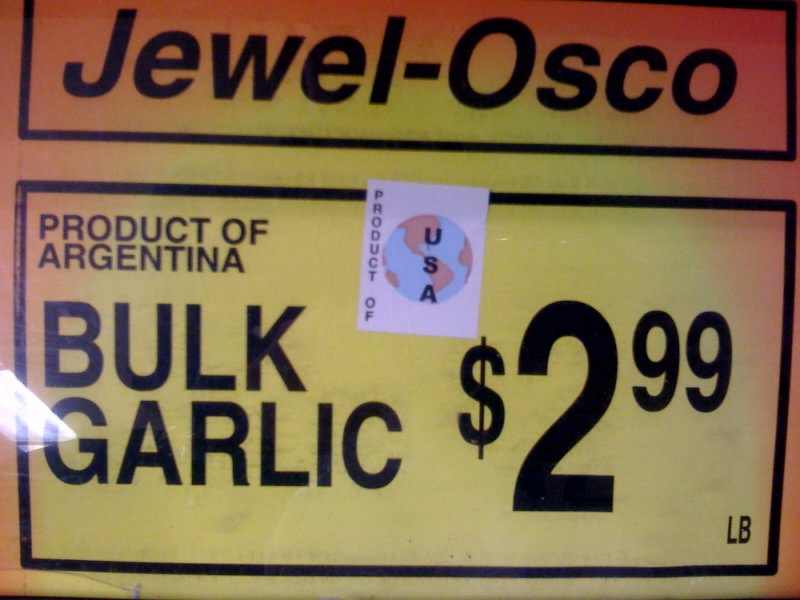This rectangular image, resembling an advertisement or a price label, features a dynamic yellow-to-orange gradient background that transitions from darker orange at the top corners to a more vibrant yellow as it moves downward. At the very top, encased in a black-lined box, the text reads "Jewel-Osco" in italicized black letters. Below this, there is a larger rectangular section highlighted by a black border with a yellow background. This section contains multiple lines of black text that read: "Product of Argentina," "Bulk Garlic," and "$2.99 per pound (lb)." Additionally, to the left of this box, there is a white sticker with a depiction of the Earth in blue and peach hues, adorned with the words "Product of" in vertical black text beside the globe and "USA" horizontally across the globe. The juxtaposition of the "Product of USA" sticker against the "Product of Argentina" label adds an element of confusion, but strongly suggests a price display for garlic that might be placed on a counter or a shelf.